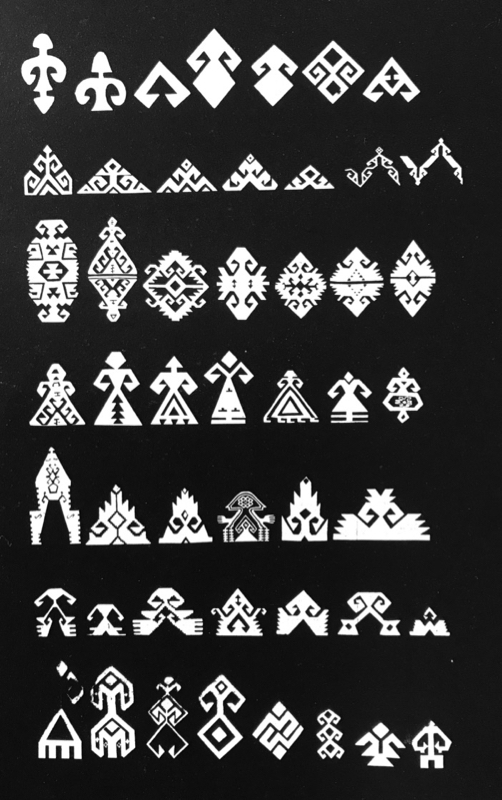The image features a series of intricate, geometric symbols, organized in seven distinct rows against a completely black, rectangular background that is taller than it is wide. The symbols are all rendered in white, creating a striking contrast. 

In the first row, there are seven symbols characterized by sharp points on both top and bottom, with arches that curl inward towards the center. The second row, also with seven symbols, showcases triangular shapes with internal patterns that curl back in a zigzag or squared-off fashion, resembling intricate pyramids. The third row continues the geometric theme with symmetrical shapes that mirror the top and bottom, featuring jagged and pointy edges. 

The fourth row presents shapes that are vaguely humanoid, particularly reminiscent of women in dresses, with wide triangular bases and arms curling inward. The fifth row includes symbols that evoke the appearance of flames, spaceships, or rockets. Moving to the sixth row, the shapes are somewhat pointy with squared-off tops, often depicting either hands or wings. Finally, the seventh row diverges with a variety of diamond and triangle shapes, some with branched parts at the bottom, and contains eight symbols.

Overall, the intricate black and white drawings exhibit a variety of shapes, from swirling and curling forms to those resembling people, keys, and trees, creating a visually complex and decorative scheme.